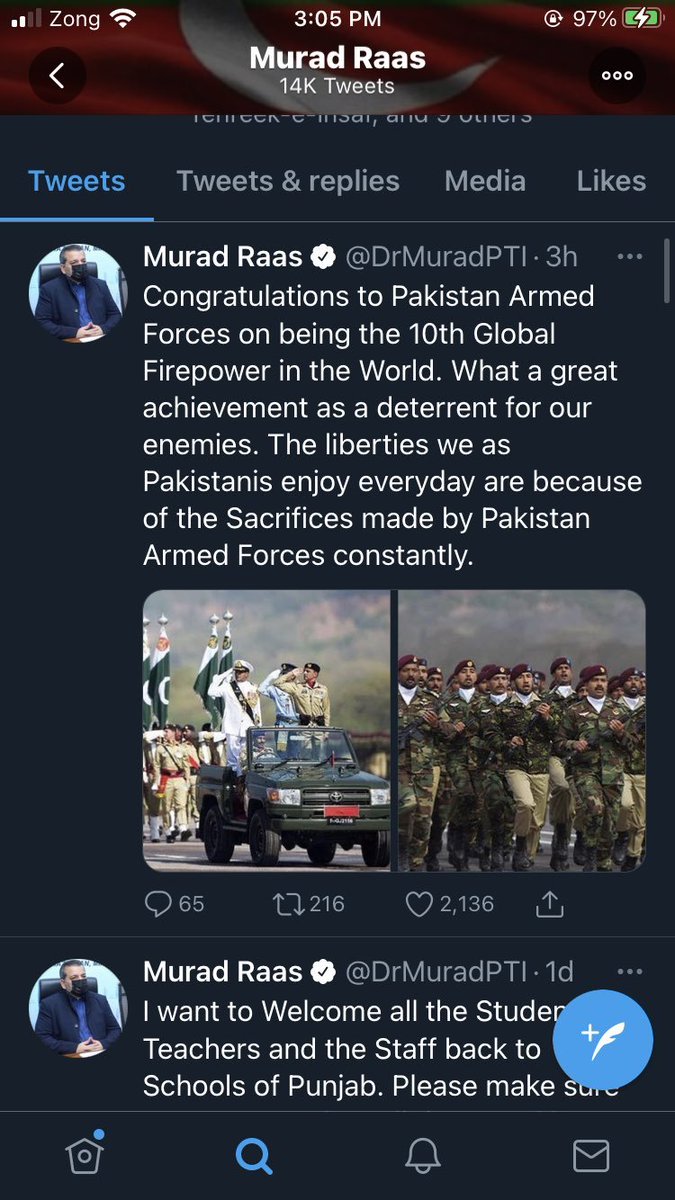**Descriptive Caption:**

A screenshot of a Twitter profile named Murad Ross, displayed on a smartphone. The phone's interface indicating the time (3:05 PM), signal strength, Wi-Fi connection, and battery status (charging at 97%) is visible along the top. The Twitter app is set to night mode, with a dark blue background and various tabs including Tweets, Tweets & Replies, Media, and Likes. The active tab is "Tweets," highlighted in blue. 

Murad Ross's profile features a background image with a flag and a verified checkmark next to his handle, @DrMuradPTI. Two tweets by Murad Ross are displayed: 
1. Posted three hours ago, it reads: "Congratulations to Pakistan Armed Forces on being the 10th global firepower in the world. What a great achievement as a deterrent to our enemies. The liberties we as Pakistanis enjoy every day are becoming of the sacrifices made by Pakistan Armed Forces constantly." Accompanied by two images of soldiers marching proudly.
2. A second tweet from one day ago is partially cut off and not fully visible.

The screenshot effectively captures the pride and respect expressed by Murad Ross towards the Pakistani Armed Forces, highlighting their global ranking and contributions to national security.